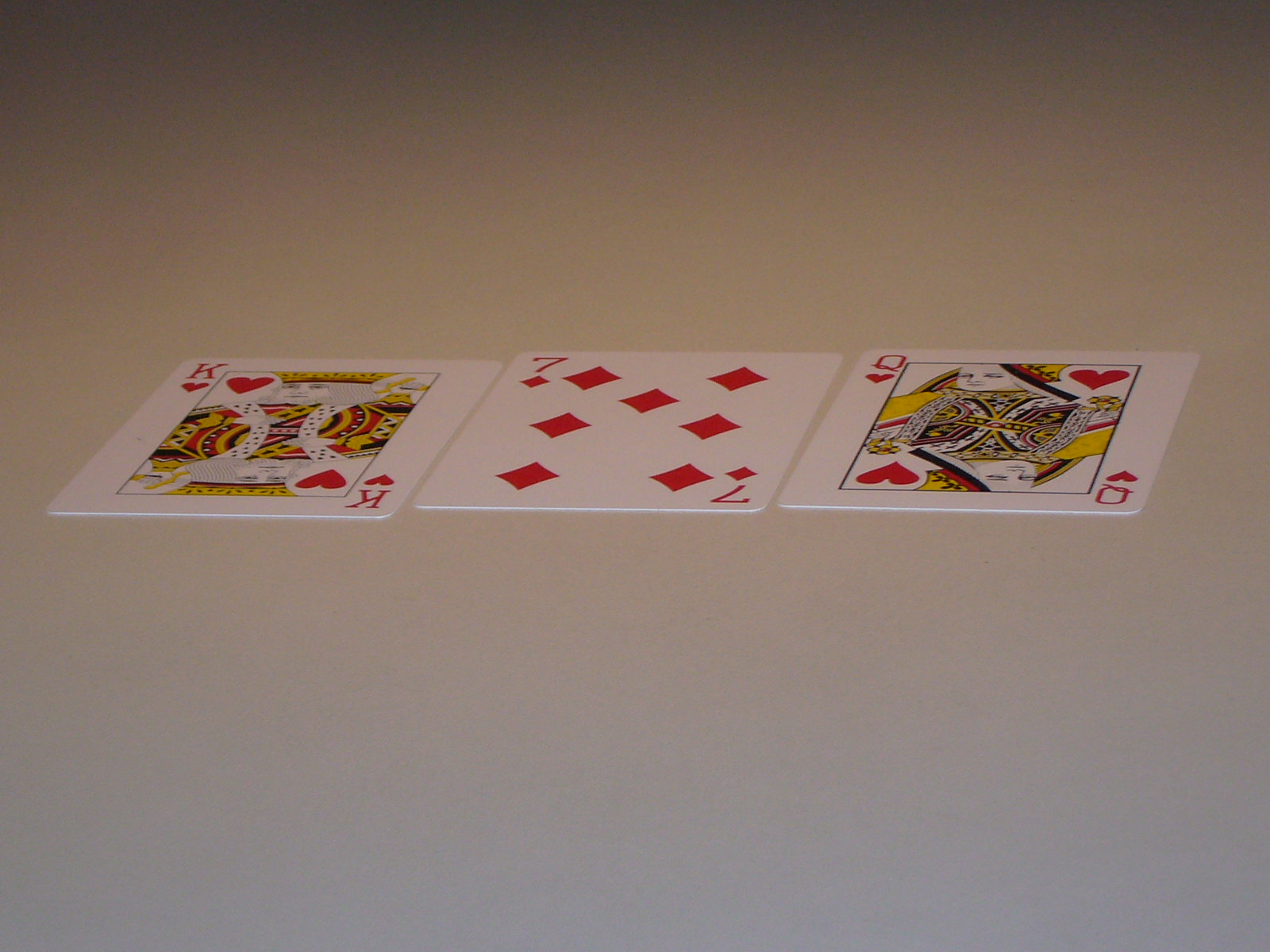In this photograph, three standard-sized playing cards are arranged on a flat, off-white surface. Distorted slightly by what appears to be a panoramic lens, the cards are stretched horizontally and compressed vertically, giving them a more square-like appearance than their usual rectangular form. The cards pictured are a King of Hearts on the left, a Seven of Diamonds in the middle, and a Queen of Hearts on the right. Each card features the traditional white face and the familiar red and black suits and values clearly visible. The background on which the cards rest is predominantly a grayish off-white, transitioning to a subtle blue hue towards the bottom of the image, and darkening somewhat at the top, likely an effect from the camera lens. This visual manipulation adds a unique artistic flair to an otherwise ordinary scene of playing cards.